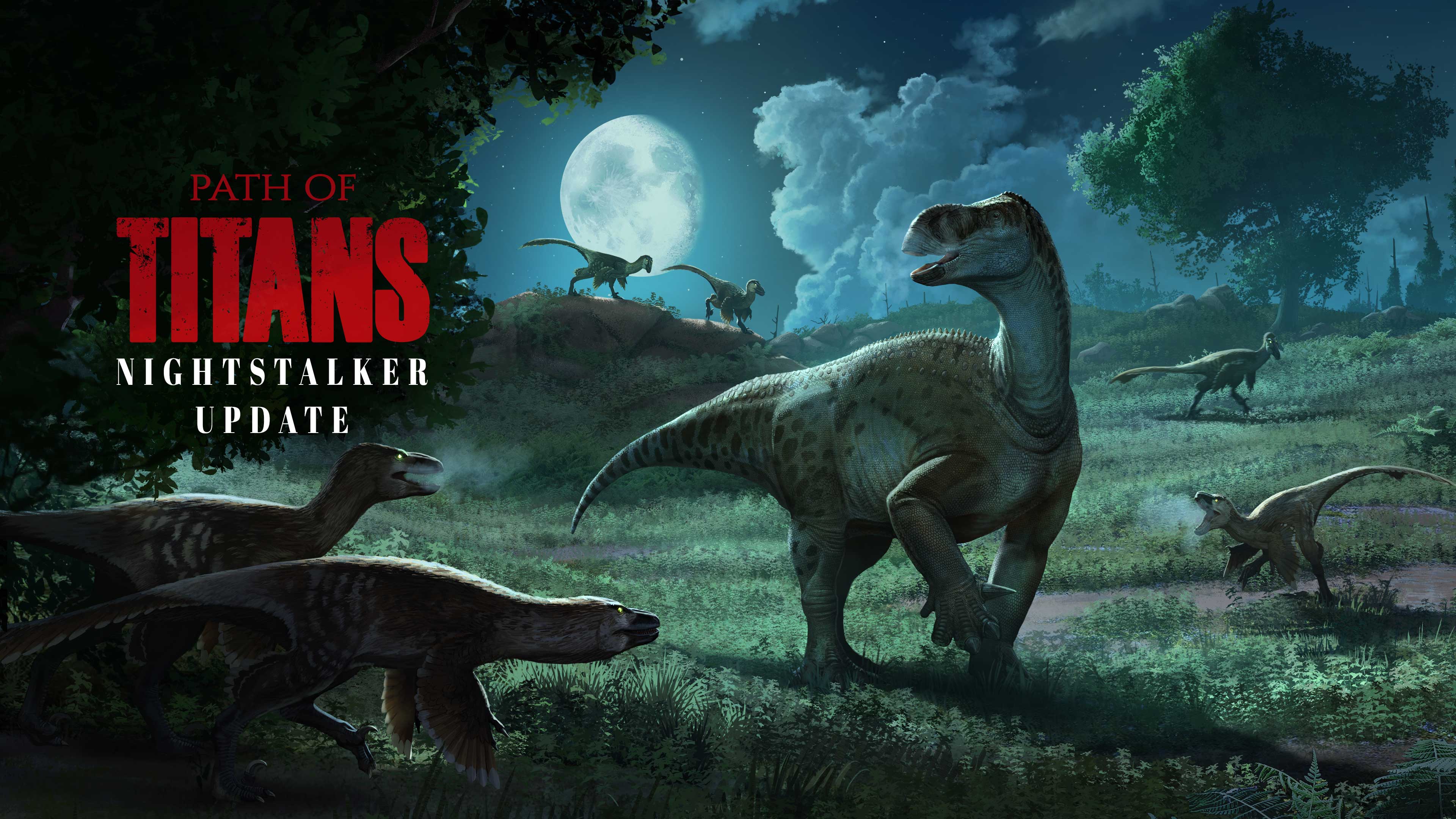The advertisement for "Path of Titans: Night Stalker Update" features an eye-catching nighttime scene, likely illustrated for a movie or a coloring book cover. Dominated by a large, full moon centered near the top, the sky is brightly illuminated, allowing for the detailed depiction of various dinosaurs. Underneath the red title text in the bottom left corner, two small theropods, resembling alligators with legs, lurk closer to their prey. The scene reveals six carnivorous dinosaurs of varying sizes cornering a single, larger herbivorous dinosaur. Positioned slightly to the right center, this stranded herbivore stands out against the white fluffy clouds and scattered green trees in the background. More raptor-like creatures are visible in the distance, descending a hill with intent. The entire setting is bathed in moonlight, making every dinosaur, patch of green grass, and shadow discernible against the dark yet vividly colored landscape of blacks, greens, blues, grays, and beiges.